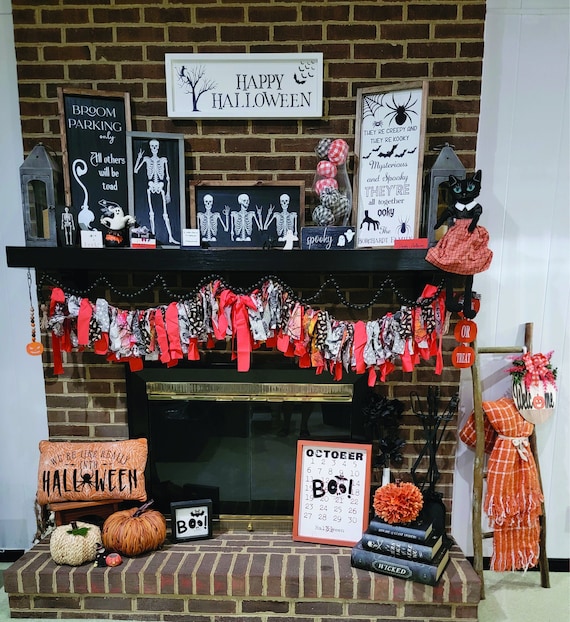The image showcases a brick fireplace and hearth elaborately decorated for Halloween. Centered above the fireplace is a white sign with "Happy Halloween" in black letters, accented with a skeleton tree and bats in the upper right corner. Flanking the sign are two tall tower-like structures: one features a black cat holding a plaid bag, while the other includes Halloween-themed pictures and signs. On the left side, there's a tall picture of a skeleton, and next to it, a "Broom Parking" sign with white writing on a black background. The mantle displays a series of images, including three horizontal skeletons below the main sign. Hanging from the bottom of the mantle is a garland made of bows and possibly socks in various colors, including red and brown with white polka dots.

The fireplace structure itself is old-style, made of red brick with white mortar and featuring two glass doors trimmed in gold. In front of it, on the hearth, there are pillows that say "Halloween," a calendar marked with "October" that also says "Boo," a stack of black books, and pumpkins and gourds. To the left of the fireplace, a pillow inscribed with "Halloween" sits atop a box that says "Boo," accompanied by crafted pumpkins. On the right side, there's a decorative sign for October and Boo, a stack of books, a set of fireplace tools, and a small rack displaying a plaid dress or outfit. The festive setup even includes a decorative blanket hanging nearby, making the entire scene a creative and detailed Halloween celebration.